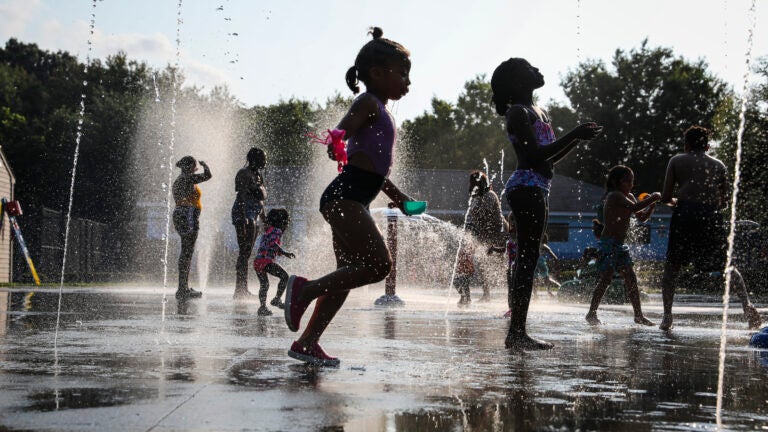In this vibrant and sunlit photograph, children in colorful bathing suits are joyously running through streams of water at an outdoor splash pad. Thin jets of water shoot up from the concrete ground, creating small puddles and a playful, misty atmosphere. Among the lively children, two young girls prominently stand in the front, while several other kids, some equipped with water guns and toys, play around in the background. A bigger fountain spray is visible in the middle, adding to the fun. Scattered among the children are adults keeping a watchful eye on the scene, standing further back, appearing as silhouettes against the bright light. The backdrop features a few buildings, including one partially obscured by the spray of water, and a fence to the left. Beyond these structures, a row of trees stretches across the horizon under a clear blue sky, dotted with a few white clouds, indicating a likely hot and splendid day.